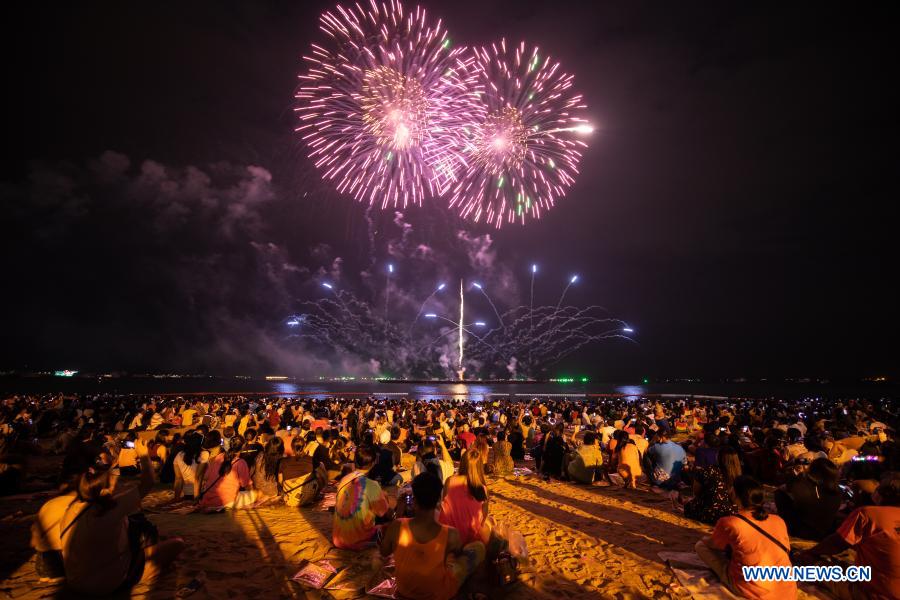A photograph captures a vibrant scene of people gathered on a golden sandy beach at night, watching a spectacular fireworks display over the water. Shot from the back of the crowd, the image showcases individuals in an array of summer clothing, including colorful tank tops and t-shirts. They sit or lounge on beach towels, all facing the midnight blue sky. Dominating the center of the photograph are two large, dandelion-shaped fireworks bursting in hues of pink, white, and orange. The black water below them reflects the mesmerizing lights. Alongside, ten smaller blue fireworks are seen ascending towards the sky, with a single column of white light shooting upwards from the ground, adding to the dazzling array of colors and shapes illuminating the night.